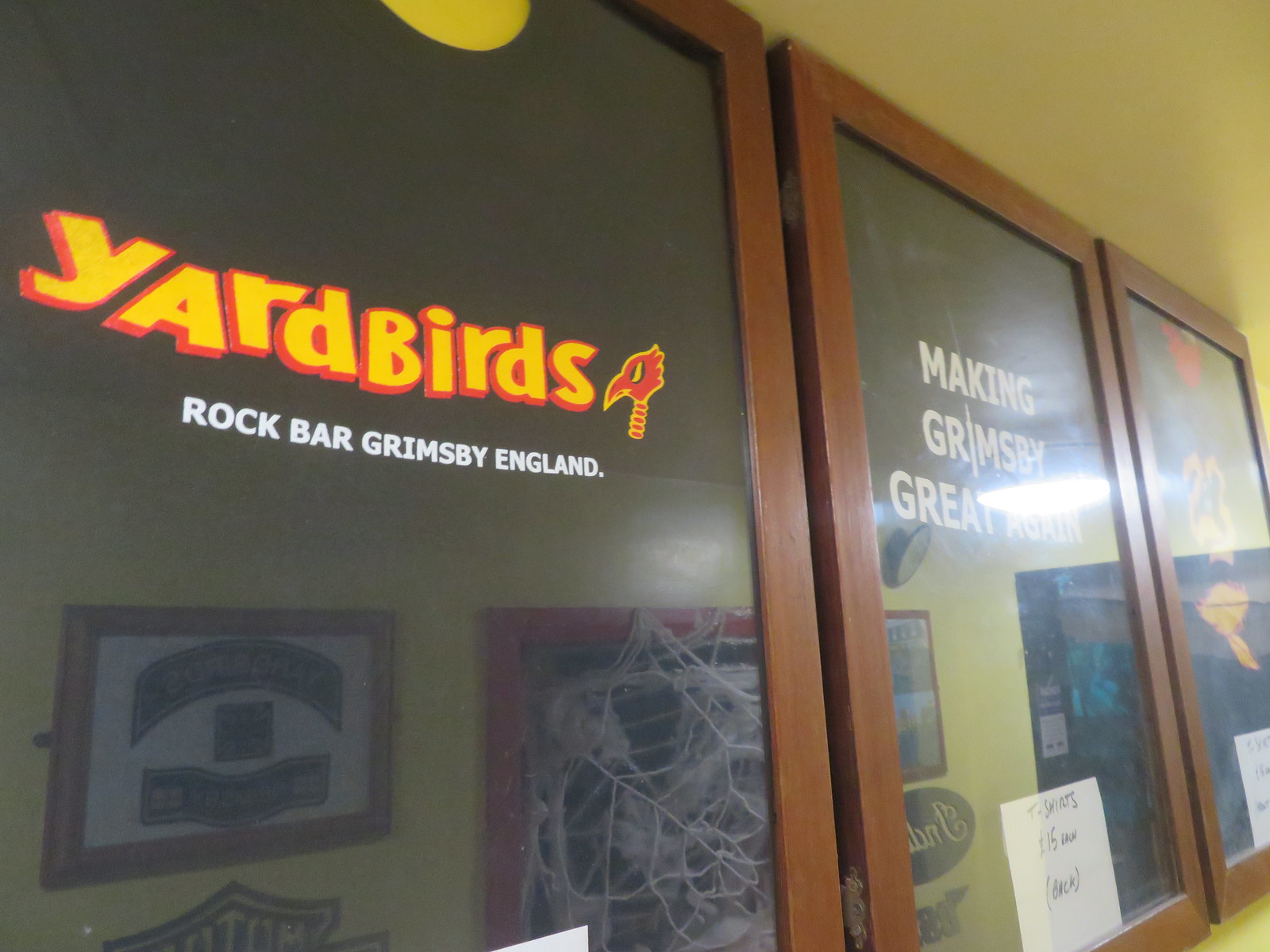The photo depicts a beige-colored wall adorned with three framed posters or signs. These glass-fronted displays possibly double as windows or doors, bordered in wood brown trim. Starting from the left, the first poster has a black background with bold yellow letters outlined in red reading "Yardbirds," accompanied by a cartoon image of a red bird’s head resembling a cardinal. Beneath in white text, it states "Rock Bar, Grimsby, England." The second poster features the slogan "Making Grimsby Great Again" in white text, with a paper taped below it announcing "T-shirts, $15 each." The third poster remains unclear due to the camera's flash and reflects several framed items from the opposing wall, including another Yardbirds plaque and a child’s art project of a spiderweb. Also visible is the photographer's faint reflection in the bottom right corner of the third frame.